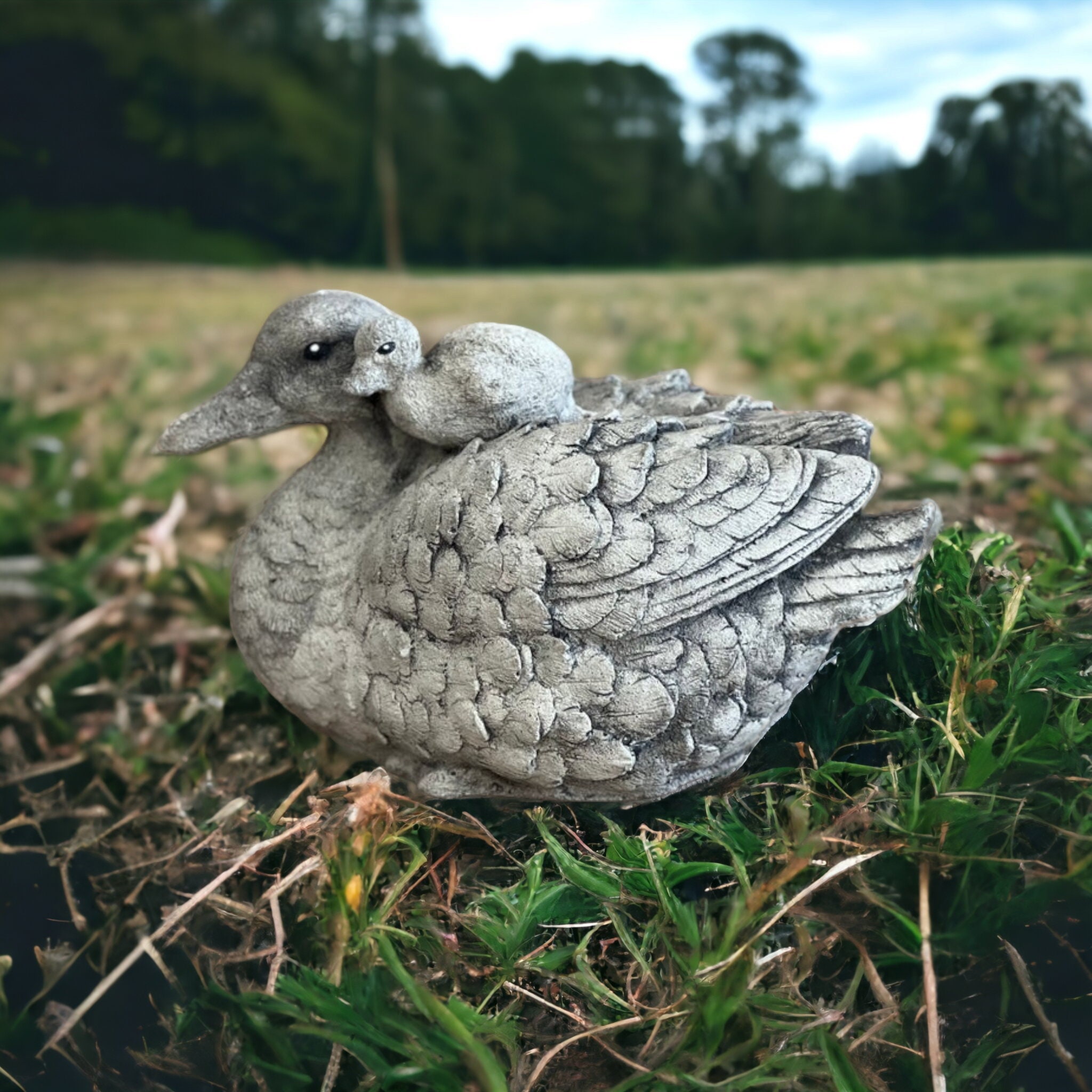In the middle of a bright, sunny day, a detailed grey sculpture of a duck and a chick, possibly made of clay, gypsum, or a similar material, sits serenely on a grassy field scattered with twigs fallen from surrounding trees. The sculpture, with intricately crafted feathers and dark gray, almost silvery edges, appears lifelike, almost mistaken for a live animal due to its texture and stillness. The duck, with its reflective black eyes, seems to gaze directly at the photographer, adding an intense, almost eerie quality to the scene. The chick, perched atop its mother, enhances the sculpture’s depiction of a tender, natural moment. The grassy field is surrounded by a blurred backdrop of thick, average-height trees, emphasizing the sculpture as the focal point in this tranquil, yet vividly alive, outdoor setting.